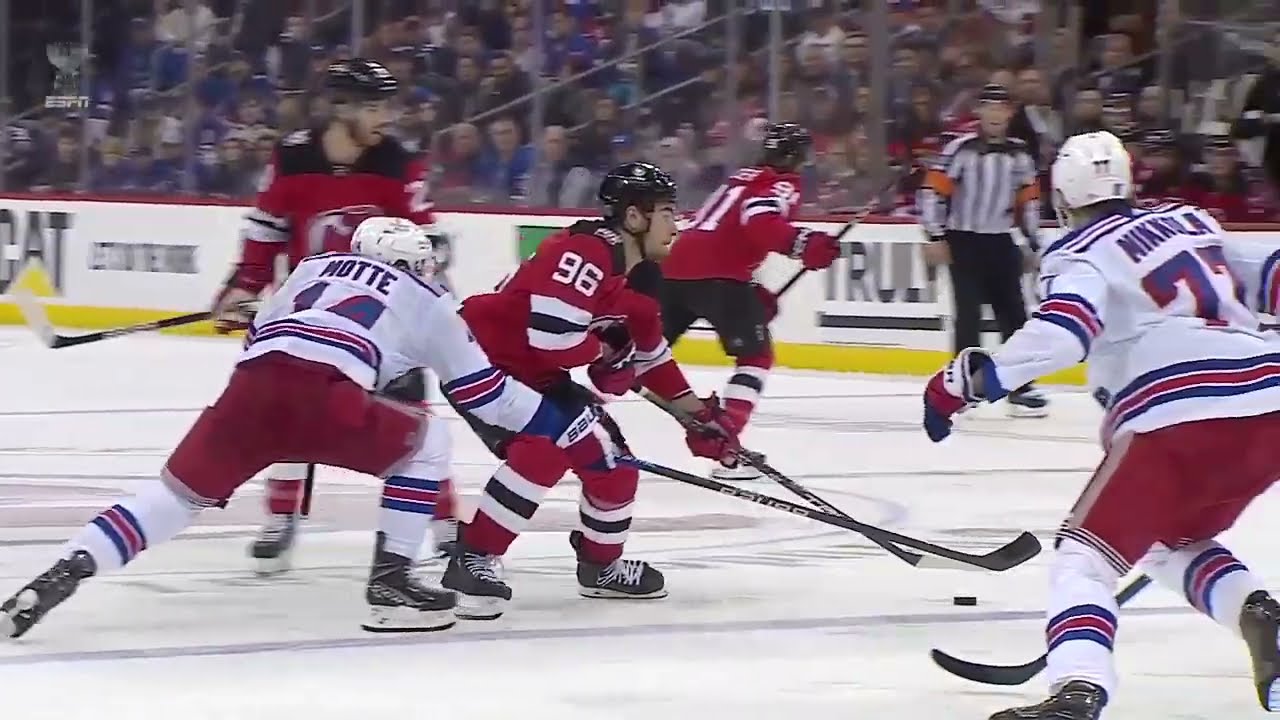The image depicts a dynamic scene at an indoor hockey game, captured from the perspective of someone standing on the ice. At the center of the action are five hockey players intensely vying for the puck. The teams can be distinguished by their uniforms: one team sports white jerseys with blue lettering, red and blue stripes, and red pants, equipped with white helmets and black skates. The opposing team wears red jerseys with white and black accents and black helmets. Among the players, two individuals in white are facing away from the observer, while two in red are side-skating towards the puck. In the background, a referee dressed in a black and white striped uniform with orange bands on his sleeves hovers at the top right, supervising the game. Above the ice, an excited crowd watches the action, separated by a protective glass and fencing. The rink is brightly illuminated, showcasing the vibrant colors of the players' uniforms—white, gray, blue, red, pink, orange, green, and yellow—against the icy floor. No readable text is present in the image, except for some partially visible words on a wall, hinting at advertisements.